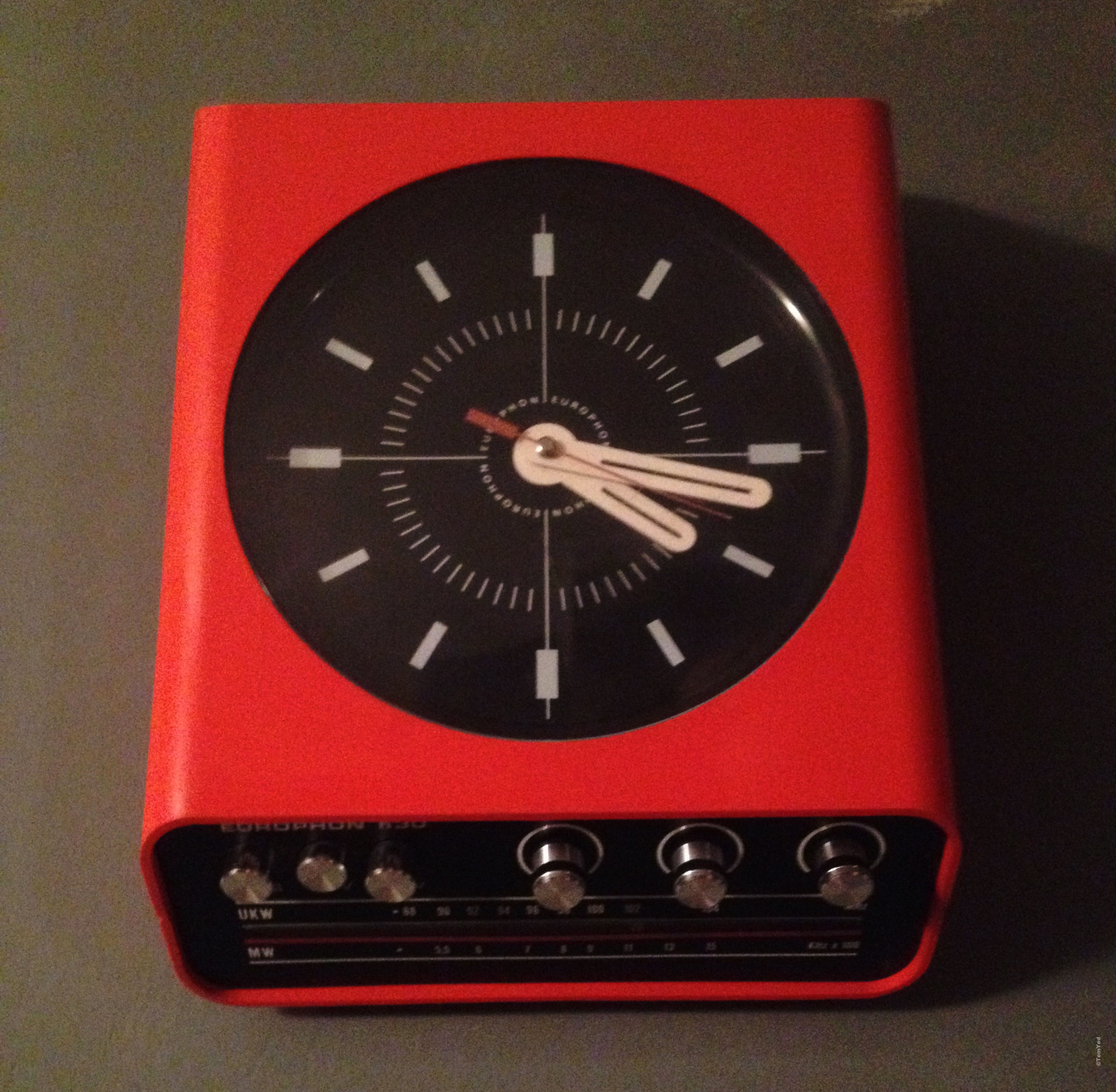The image depicts a bright red radio clock device with a futuristic appearance. The top of the device features a black clock face without numbers, replaced instead by white dashes forming concentric circles. The hour, minute, and second hands point to approximately 5, between 4 and 5, and 18 minutes past, respectively, with the second hand being red. This clock component is encircled at the top of the device. Below the clock face, along the front of the device, are six silver knobs and buttons, arranged in two groups of three on either side, resembling controls on an old stereo. The casing of the device is red with a black backing, and it is situated on a gray surface. Although specific functions of the knobs and elements below them are unclear, there is some unreadable lettering above the knobs. The device is relatively tall and box-shaped, approximately a foot in both height and length.